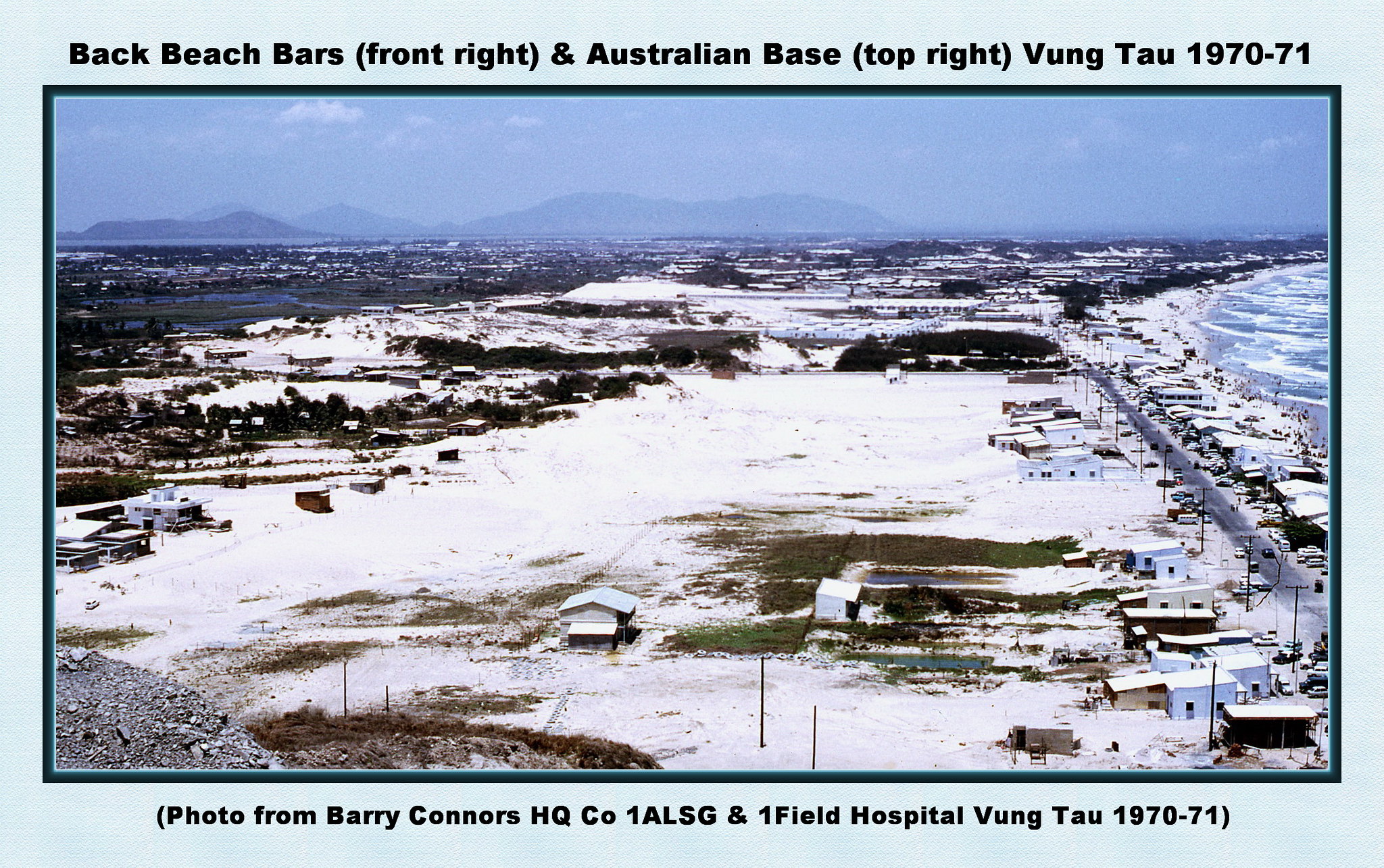This aerial photograph, bordered in light blue and green, captures a detailed snapshot of a snowy landscape in Vung Tau, circa 1970-71. The top of the photo is marked with the text "Back Beach Bars, front right, and Australian Base, top right, Vung Tau, 1970-71." At the bottom, it reads, "Photo from Barry Connors HQ Co 1ALSG and 1 Field Hospital, Vung Tau, 1970-71." The image showcases a sprawling, snowy area dotted with small houses, man-made structures, and a strip of road lined with telephone poles and scattered cars. To the right, beach waves crash against the shoreline, suggesting the presence of a body of water. In the backdrop, barely visible, are distant mountains, hinting at the cold, wintry conditions. The photograph captures an Australian base, set against a landscape that blends the pristine white of snow with patches of greenery.